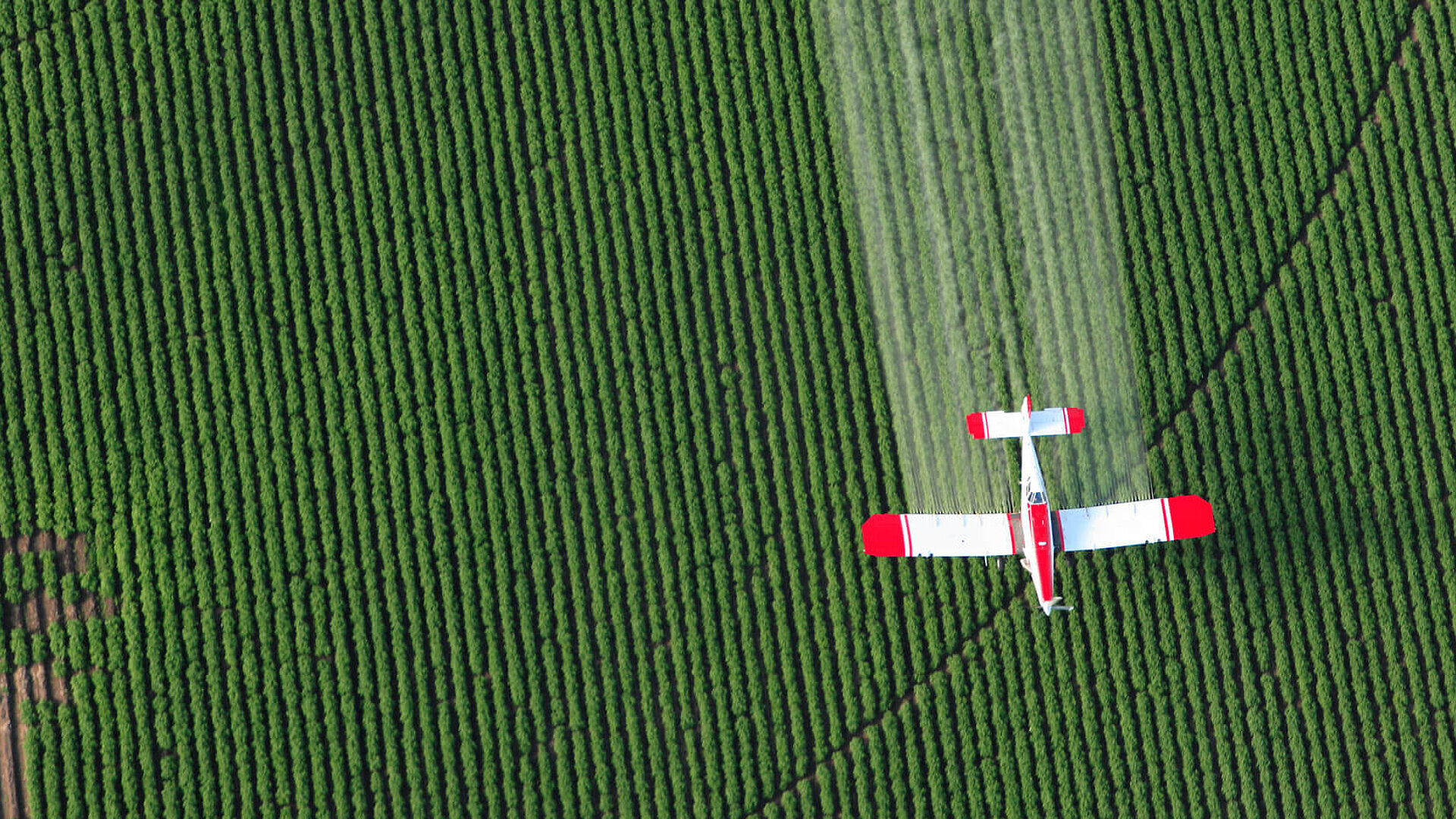This is a detailed aerial photograph of a vibrant green field meticulously planted in rows, likely crops or grass. The field features straight, uniform lines with a diagonal C-shaped path cutting through the center. There is a small, single-engine biplane flying close to the ground, easily identifiable by its white body accented with red markings on the wingtips, the back wings, and a red stripe down the middle from the cockpit to the propeller. The plane is releasing a white powdery substance, which is visible as a pale, off-white trail behind it, indicating it's likely spraying fertilizer or chemicals. Despite the field's large expanse, no people are visible. This scene contrasts the vibrant green of the crops with the stark white of the plane's spray, creating a prominent visual effect.